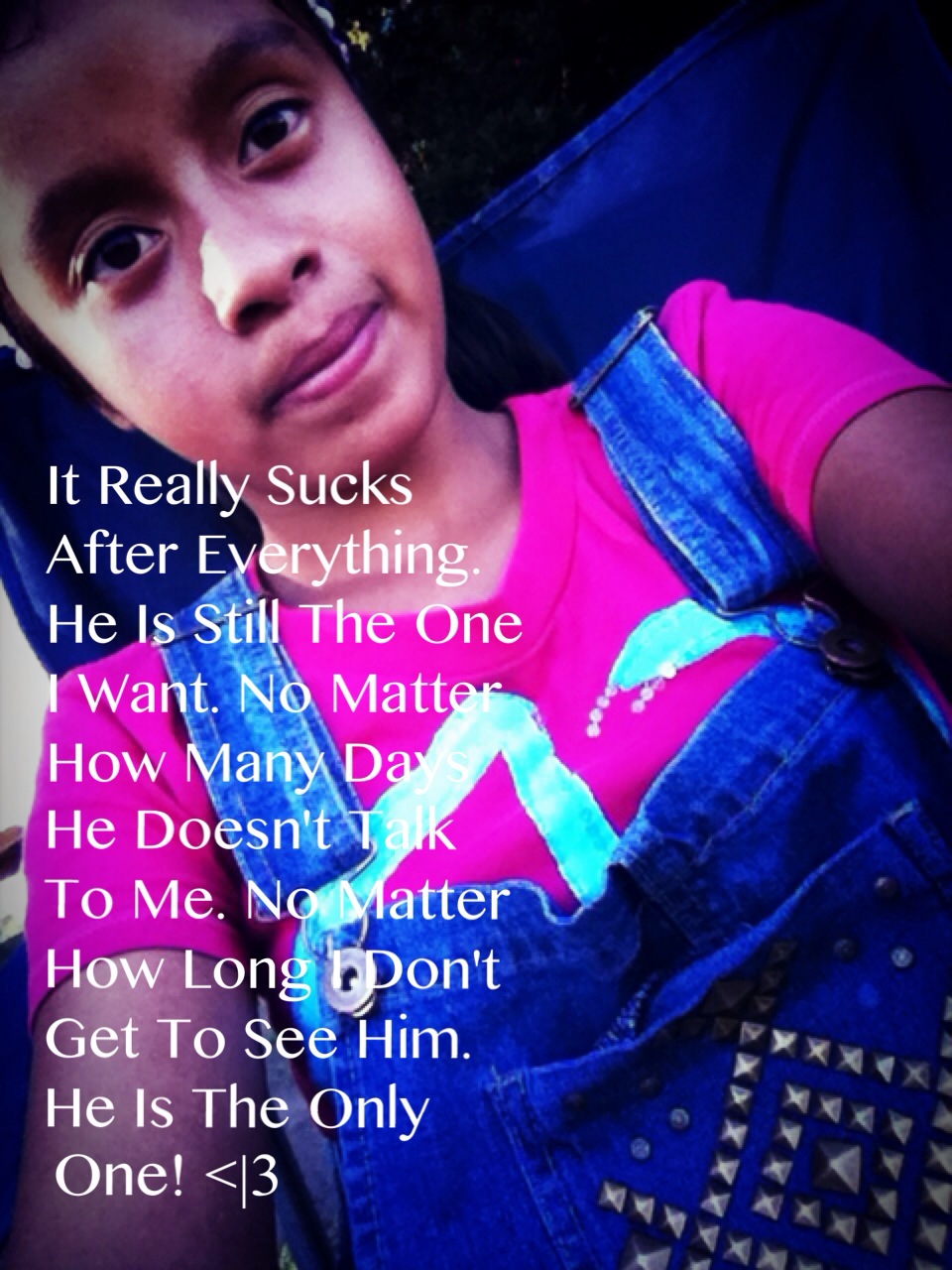This tall rectangle image features a selfie of a woman with a poignant quote overlaying it. Positioned diagonally, her head is tilted toward the top left corner, with her forehead cropped by the image's edge. Her gaze is direct, with wide-open eyes and slightly pursed lips, almost forming a half-smile. She has light brown skin and is dressed in a vibrant pink t-shirt paired with blue jean overalls adorned with patterned gold studs. The background of the photo is dark, adding to the image's somber tone. In white text over her torso, the quote reads: "It really sucks after everything. He is still the one I want. No matter how many days he doesn't talk to me. No matter how long, don't get to see him. He is the only one." Her expression and the text together convey a deep emotional longing and heartache.